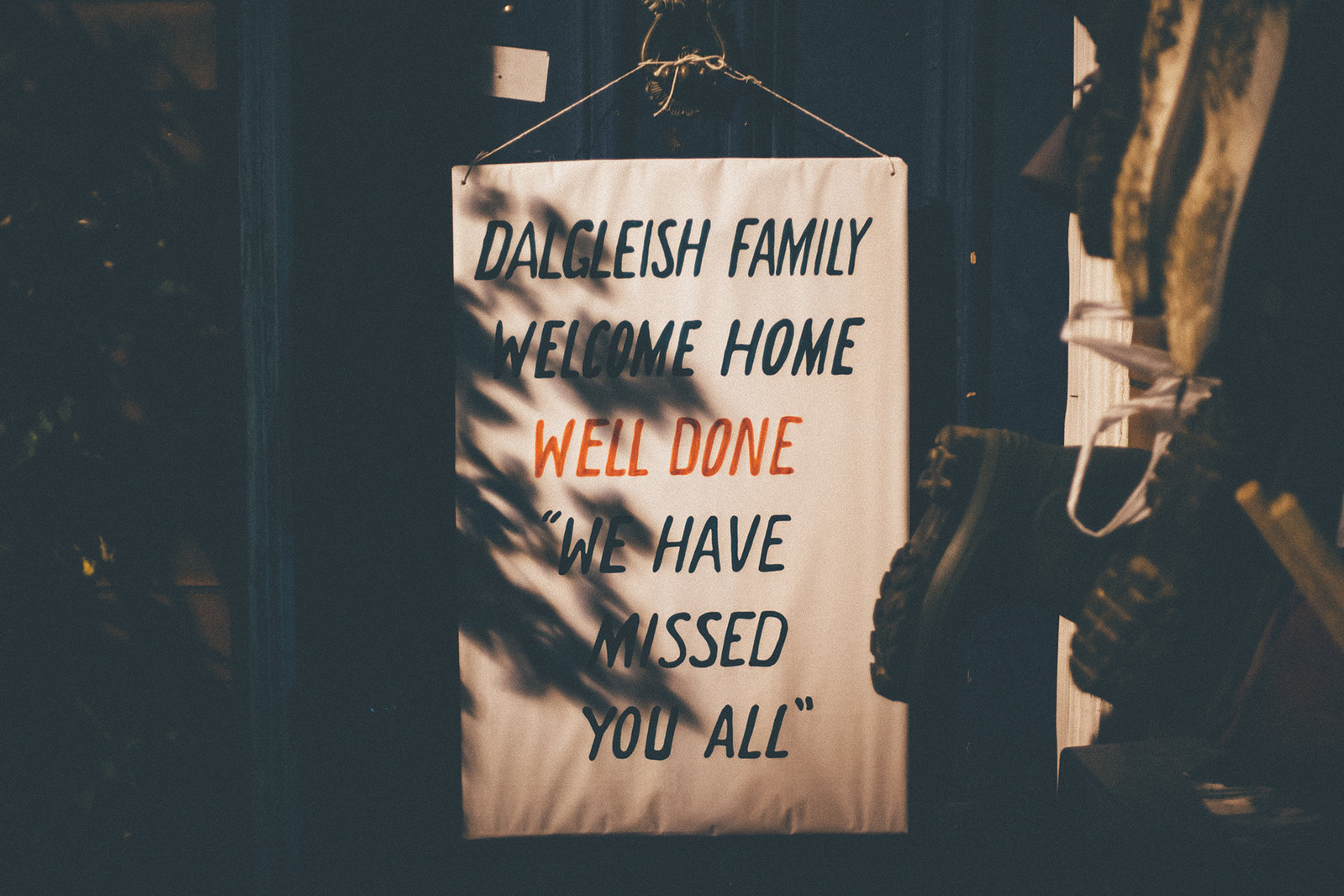The image shows a heartwarming welcome home scene for the Danglish family, centered around a prominent white banner hanging on the family's dark blue door. The banner reads, "Danglish family, welcome home, well done, we have missed you all," with the words "well done" emphasized in green. The scene is quite dimly lit, which causes details like shadows and the interior or exterior setting to be ambiguous. However, one can discern multiple pairs of boots hanging horizontally from poles to the right of the door, possibly indicating that the photo was taken in a cluttered pantry or entryway. Shadows, possibly from a tree or houseplant, slightly obscure parts of the banner. The sign and the arrangement of boots create a welcoming, albeit cluttered, atmosphere, emphasizing the family's sentiment of missing and celebrating the return of their loved ones.